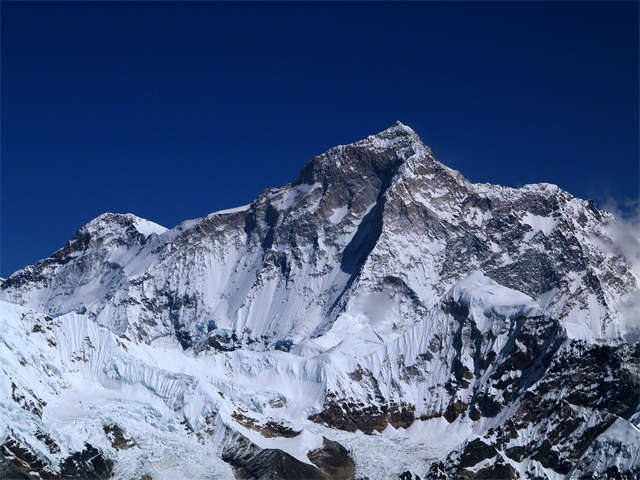This landscape-oriented photograph captures a majestic, steep mountaintop, predominantly covered in white snow with patches of dark gray rock peeking through. The mountain extends from the left to the right side of the frame and rises to a significant height, culminating in a prominent peak near the center of the image. The sky above is notably dark navy blue, almost unnaturally so, and spans the top third of the picture without any clouds. On the far right side, there is a hint of clouds or fog hugging the mountain. The rugged terrain and the absence of people highlight the mountain's raw and untamed beauty. The overall scene evokes a sense of grandeur and isolation, reminiscent of the towering peaks in the Himalayas.